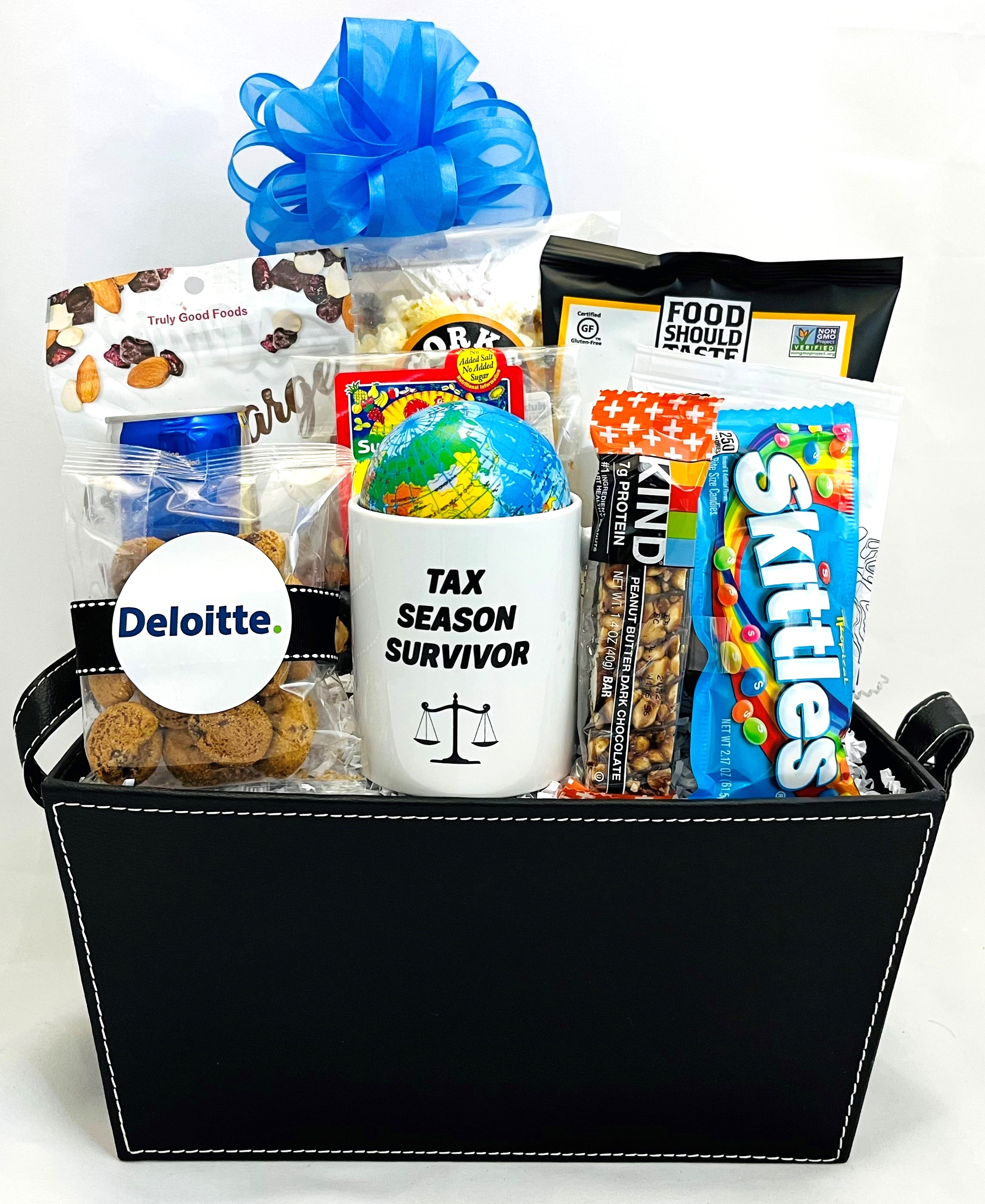This photograph showcases an intricately arranged gift basket, predominantly black with white stitching details. At the very top of the basket, a large, fluffy blue ribbon bow stands out. Centrally positioned within the basket is a white coffee cup that reads "Tax Season Survivor" in black text, adorned with a design of hanging scales of justice. Inside the cup, there is a little ball resembling a globe. Surrounding the cup, the basket is filled with a variety of treats. On the left side, there's a plastic Ziploc bag labeled "Truly Good Foods," featuring images of almonds and raisins, next to a mini bag of chocolate chip cookies with a Deloitte banner. Adjacent to these, there's a package of popcorn. The right side houses a blue bag of Skittles candy and some peanut butter dark chocolate candy bars. Additionally, there are more snacks partially visible in the background, indicating an assortment of culinary delights. The entire ensemble of treats is nestled within what looks like canvas or a lined box, all resting atop a possible stuffing material to elevate and display the items attractively.